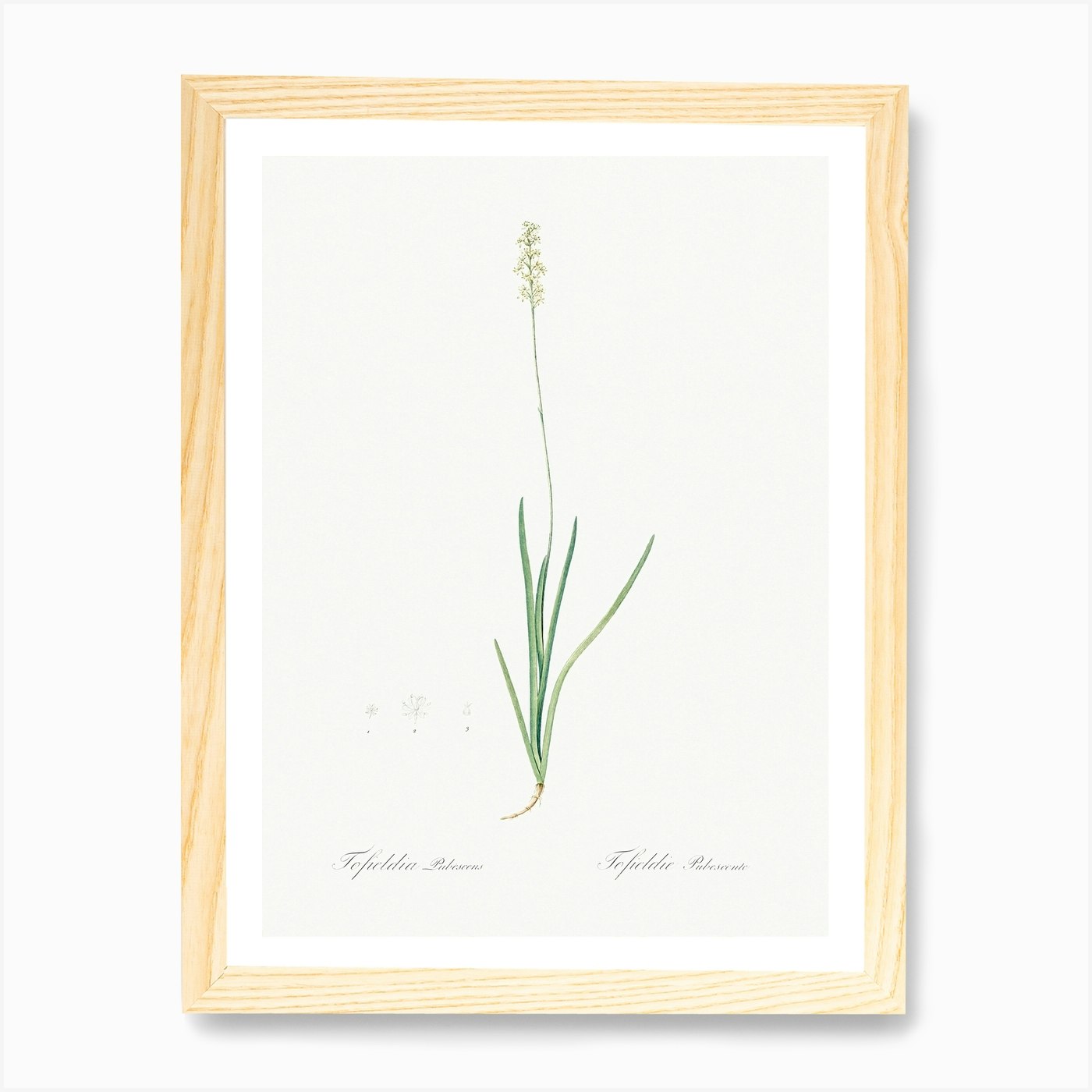This detailed image is a digital representation of a painting, possibly a computer-generated graphic with a lifelike appearance. The painting is enclosed in a light brown wooden frame with a white mat and an off-white background. It features a delicate flower on a very thin, tall stem, showcasing either small white or yellow petals. The flower is accompanied by five long, grass-like green leaves extending slightly outward from the base, with whitish-brown roots visible below. The name of the flower is inscribed at the bottom in black script, but the text appears faint and is difficult to decipher. The primary colors in the image are white, green, and brown. Overall, the image depicts the intricate details of a small, delicate flower highlighted by its naturalistic framing and subtle color palette.